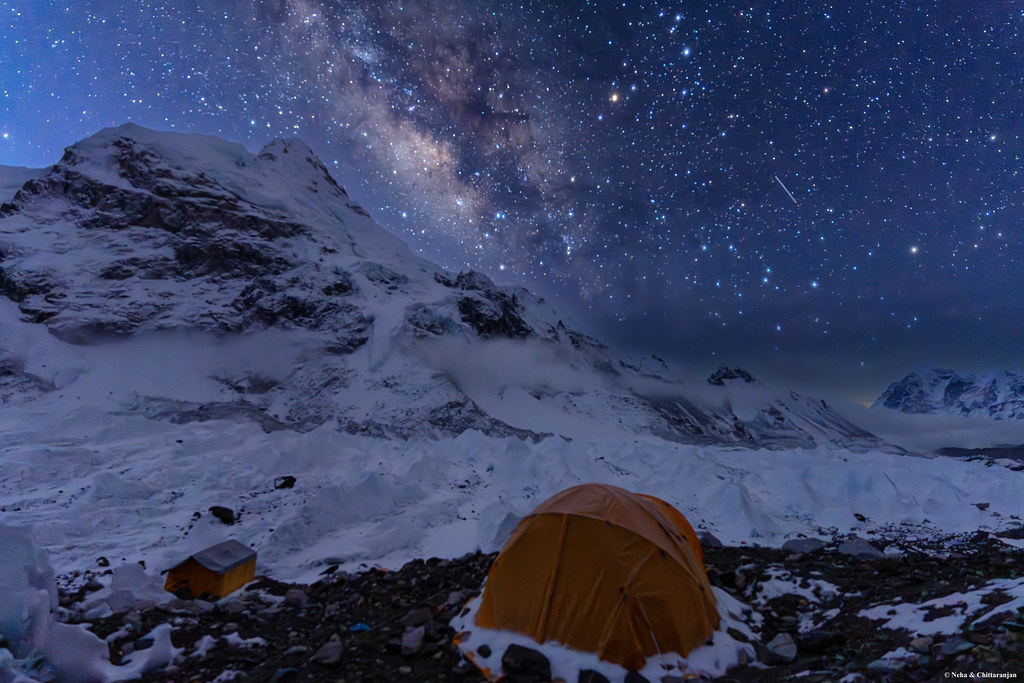This outdoor image captures a remote, snowy mountain landscape under a dark navy blue night sky filled with countless stars. The scene includes two prominent orange tents: a dome-shaped one situated atop the rocky, snow-covered mountain, and a larger, rectangular tent at the base, resembling the shape of a house from afar. Thick snow blankets the foreground, adding to the scene's cold, rugged atmosphere. The crisp night air is subtly illustrated by a faint smoke or vapor rising at the base of the mountain. A watermark at the bottom right corner credits "NIHA and Chiatarjan," adding an official touch to this striking depiction of a serene yet harsh winter night in the wilderness. The overall color palette emphasizes the dark blue and gray hues that convey the chill and isolation of the setting.